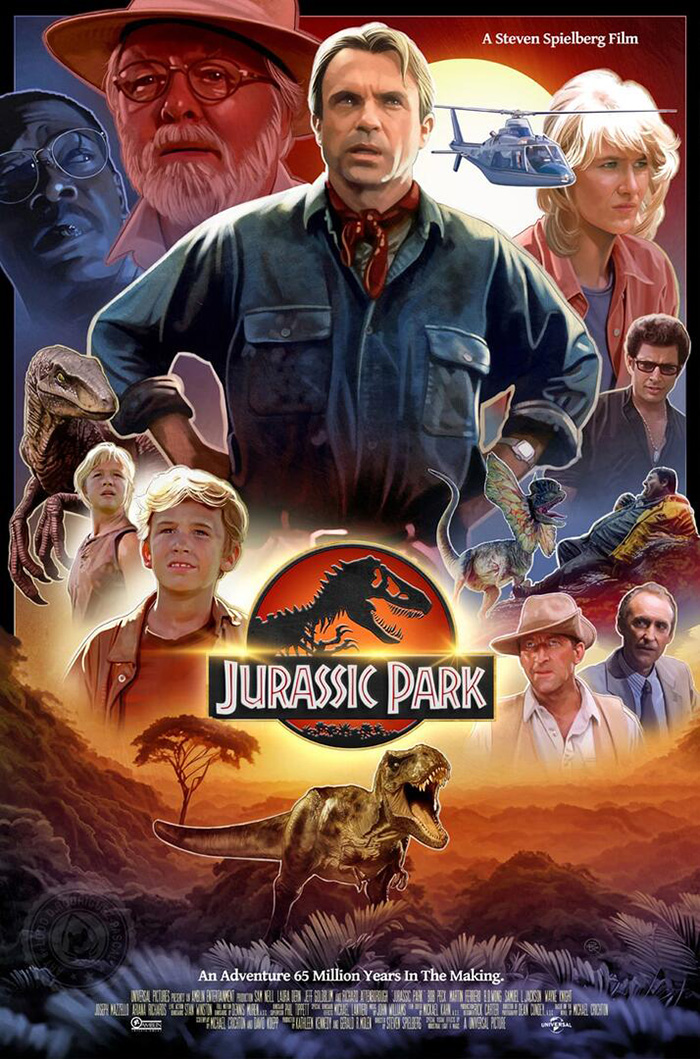The image is a detailed poster for the movie "Jurassic Park." Central to the poster and slightly towards the bottom is the iconic Jurassic Park logo, featuring a dinosaur skeleton set against an orange sunset background. The logo text is white with a red stripe and outlined in black. Below the logo, a ferocious Tyrannosaurus Rex roars, its head pointing forward and its tail to the left, standing amidst rugged terrain with bushes and a single tree.

Above the logo, the main characters are prominently displayed. Standing with his hands on his hips is a man in a blue long-sleeved shirt and red bandana around his neck. To his right, a helicopter hovers over his shoulder, and nearby is a blonde-haired woman. To his left, an older man with a white beard wearing a hat and glasses is seen. In the upper left corner, another man with round glasses, possibly in his 30s or 40s, is visible. Scattered around the poster are smaller images of other characters from the film, enhancing the sense of adventure. Text at the bottom of the poster reads "A Steven Spielberg Film" and "An Adventure 65 Million Years in the Making," and the credits are also visible. The entire composition encapsulates the thrilling essence of the movie "Jurassic Park."